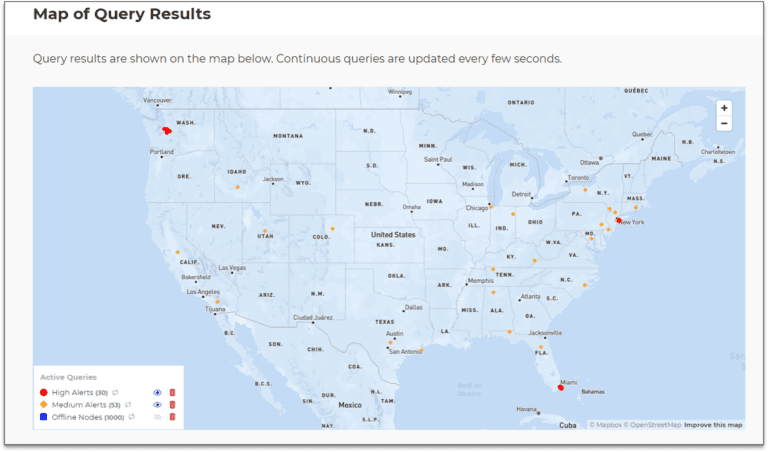This image features two maps that provide a detailed visualization of query results. The smaller map at the top displays the outcomes of written queries, which are continuously updated every few seconds. Below, the larger map shows an array of colored dots in red, yellow, and blue, each representing varying alert levels. An accompanying key highlights the following alert statuses: high alerts (30 active queries), and medium alerts. The comprehensive layout not only indicates the real-time query results but also prioritizes alerts based on their urgency.